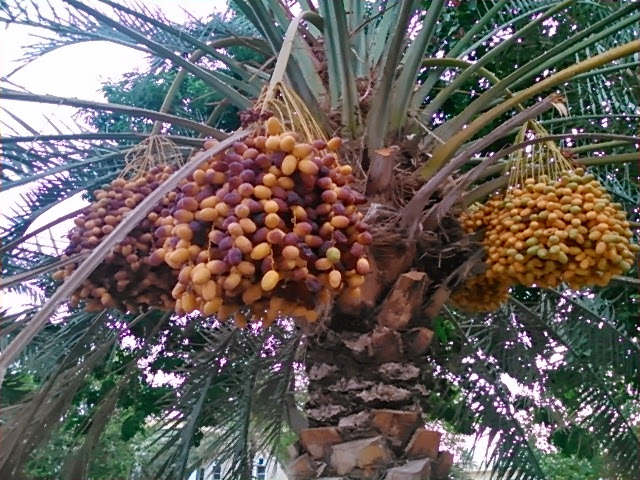The image captures a majestic date palm tree, characterized by its sturdy trunk adorned with brown prune stubs. The tree's verdant fronds create a lush canopy, from which clusters of date palms dangle. There are four to five bunches of date palms, which exhibit a mix of yellow and brownish hues, adding a vibrant contrast to the green leaves. The photograph's perspective looks upwards from the base of the tree, emphasizing the tall and robust nature of the palm. The setting is outdoors under bright sunlight, enhancing the clarity and vividness of the scene. The background features a clear sky and nearby trees, contributing to the natural ambiance. The palm tree stands upright with its textured bark and multiple branches, showcasing both ripe fruits and elegant greenery, indicative of its mature and enduring presence in the landscape.